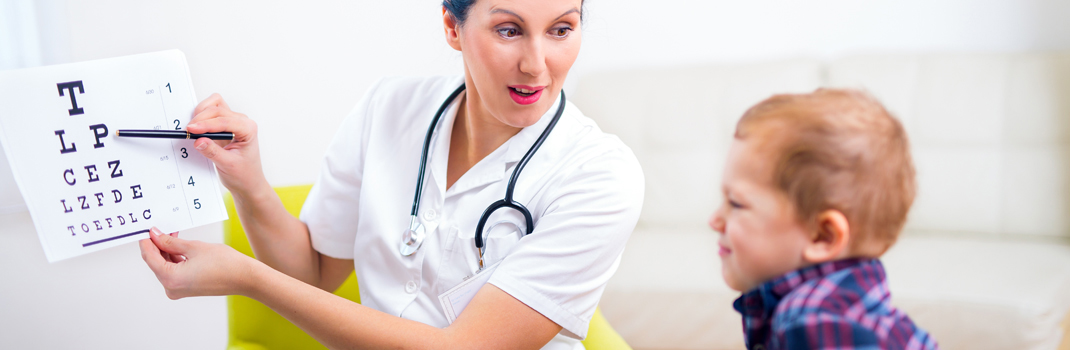In this detailed photograph, a female medical practitioner, possibly a doctor or nurse, is seen administering an eye exam to a small child. The setting appears to be a comfortable medical office, though the background, including a white couch, is slightly out of focus. The woman's dark hair frames her face as she focuses intently on the task at hand. She is dressed in a professional white buttoned-up medical shirt with a front pocket, and a stethoscope with black wiring is draped around her neck.

She holds an eye chart prominently in her left hand, displaying a series of letters: T-L-P-C-E-Z-L-Z-F-D-E-T-O-E-F-D-L-C. Using a pen, she points to the second line of the chart, specifically to the letters "L-P," guiding the child through the vision test. The child, wearing a blue and purple plaid shirt, is engaged in the activity, squinting slightly and looking towards the chart. His body is turned to the left, indicating his concentration on identifying the letters shown to him. The intimate and professional setup highlights the careful interaction between the caregiver and the young patient, emphasizing the nurturing environment of the medical examination.